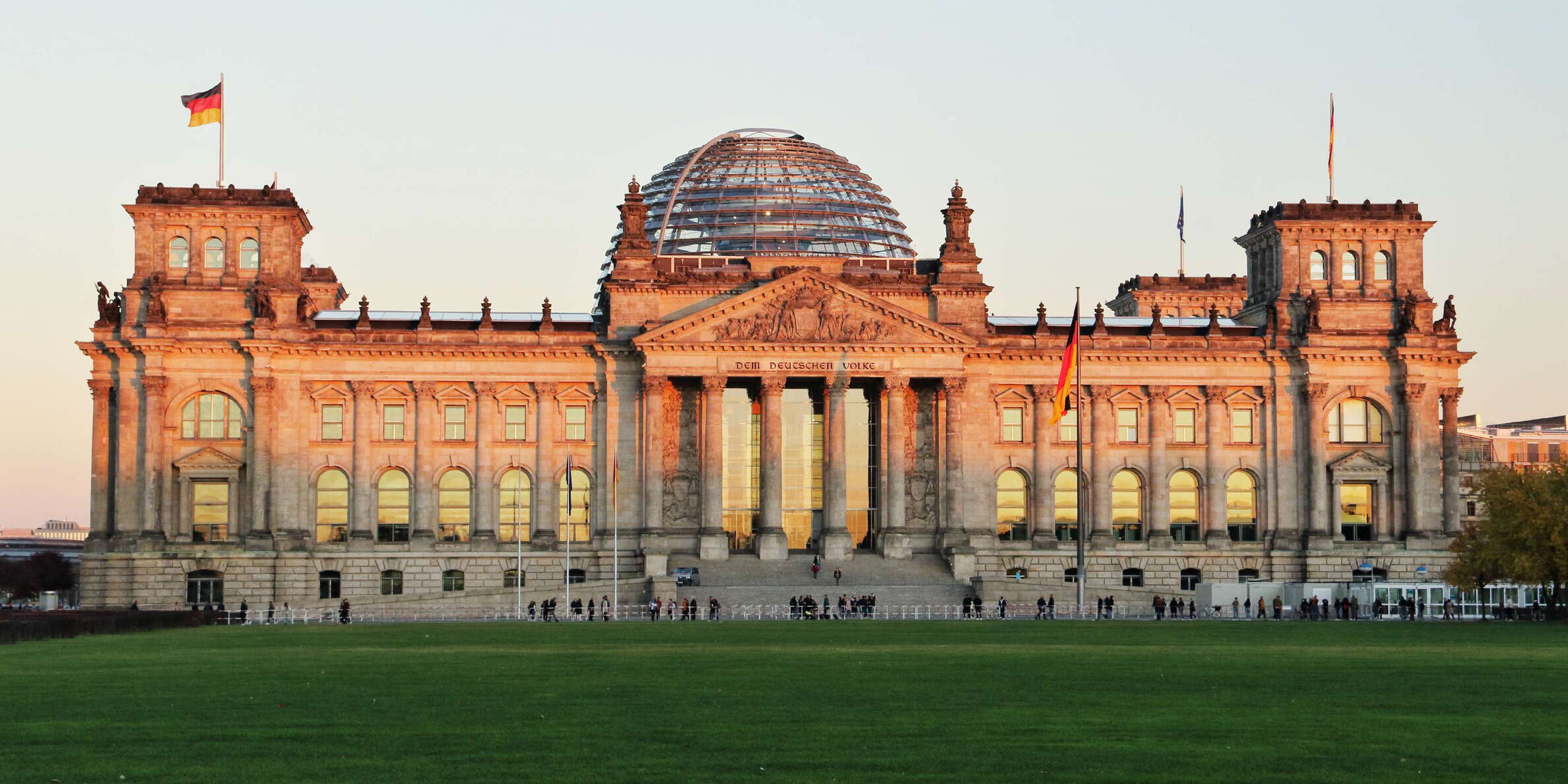The photograph captures a grand neoclassical building, likely of political significance, situated in Germany. This deduction comes from the presence of German flags—the iconic black, red, and yellow tricolors—one of which is prominently displayed on the top left-hand side of the building and another larger one positioned on the ground at the front right. The building's architecture is characterized by its seven imposing columns at the main entryway, flanked by at least five archways on either side and additional corner archways on both ends.

The structure features at least three stories, with two primary levels above ground and possibly one subterranean level accessible via the entryway stairs. The front facade is adorned with statues that resemble solemn figures rather than grotesque gargoyles, adding to the ornate and classical appeal. Notably, a distinctly modernist dome made of gray metal and glass rises from the center of the building, encased in a coppery wireframe that contrasts with the otherwise traditional aesthetic.

Set against a backdrop of a gradient sky that transitions from a pinkish hue near the horizon—reminiscent of sunrise or sunset—to a more subdued gray-blue further up, the scene is bathed in a serene light. The expansive, well-manicured lawn in the foreground leads up to a short white fence and broad steps that welcome visitors. Small groups of people can be seen walking around and ascending the steps, highlighting the building's probable status as a significant and possibly touristic landmark. The structure's color palette transitions from a brick red at the top to a gray stone or cement lower down, hinting at a blend of materials and hues that complement its historical and architectural grandeur.